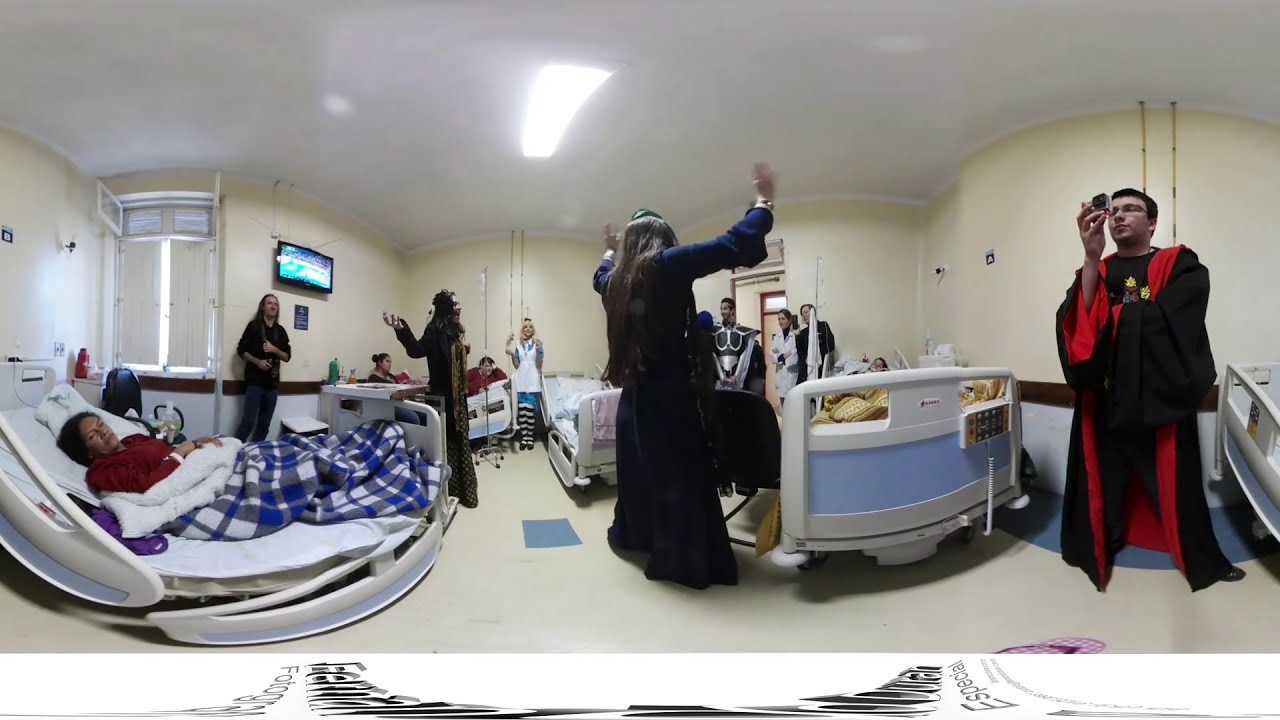The image depicts a wide panoramic view of a hospital room. Dominating the scene are two white hospital beds with blue trim, each covered with differently colored blankets—gold for the unseen patient on one side and various other colors for the other beds. The room is pristinely white, with both the floor and walls matching in color, and it features medical monitoring technology on each side. A dark-haired woman in a maroon gown occupies one of the beds, while a TV is mounted on the wall near the ceiling.

The photo captures a lively event aimed at cheering up the patients, possibly a cosplay or Halloween celebration. Various individuals are dressed in character costumes, including Alice from Alice in Wonderland who stands out distinctly. In the middle of the room, a woman dressed in a blue costume raises her hands as though partaking in a performance. Multiple people in the room, at least two on each side of the beds, are wearing costumes that include Harry Potter characters and a black-robed wizard. These costumed individuals appear to be engaging in some sort of ceremonial or uplifting activity for the patients. The overall atmosphere in the image is one of encouragement and festivity amidst the clinical setting.